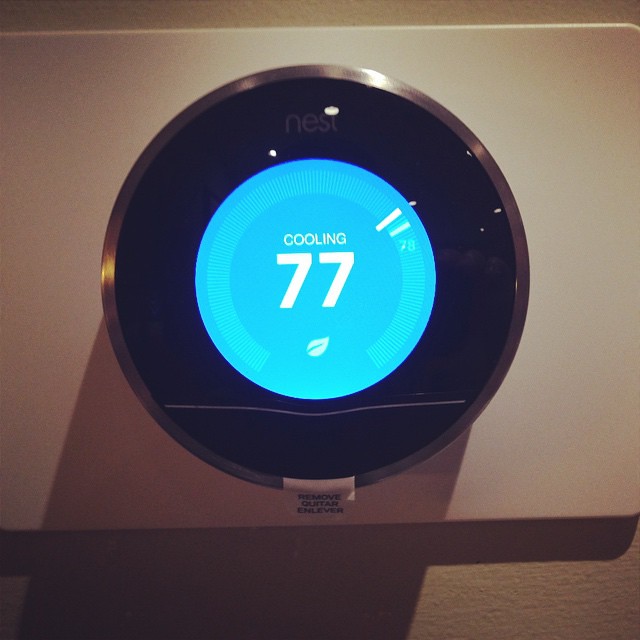The image depicts a circular, pewter-rimmed thermostat mounted on a plain white wall. Due to the camera angle, the device appears somewhat dark. The thermostat is encased in a bracket with visible instructions to "remove" something written in multiple languages, though the tab hasn't been removed yet. Surrounding the thermostat's face is a wide black band, marked by what seems to be a scratch at the bottom.

At the core of the thermostat, shades of blue and green dominate. The blue forms an incomplete border around a central green section, both of which are marked with small slashes indicating temperature readings. The display shows a current cooling temperature of 77 degrees and features a small leaf symbol near the temperature reading, the purpose of which remains unclear.